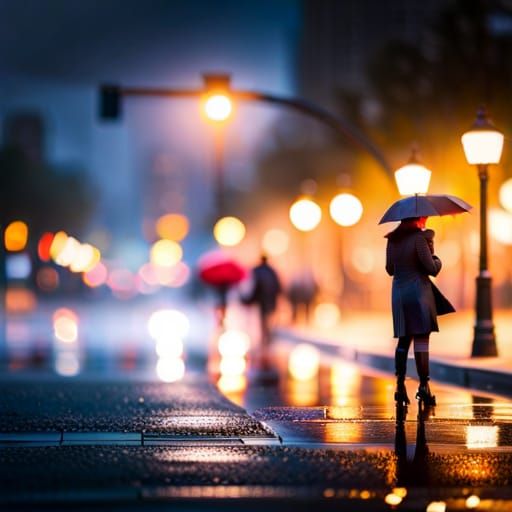A detailed and descriptive caption combining elements from the three provided captions:

"This image, likely AI-generated due to its smoothness, depicts a rainy night scene on a bustling city street. The background is intentionally blurred, highlighting colorful, out-of-focus lights in hues of orange, blue, red, white, and pink. Blurry buildings and pedestrians add to the city's lively atmosphere. The main subject, a woman standing on the right side of the road, wears high-heeled dark boots and a black coat. She holds a gray umbrella, protecting herself from the rain as the wet street below her reflects the city lights. Several tall lanterns or gas lamps line the sidewalk she stands on, cutting into the blurred background. A yellow street light and a blurry traffic signal hover above, casting a vivid glow. Raindrops and their reflections on the glossy surface indicate the ongoing downpour, enhancing the melancholic yet vibrant night setting."